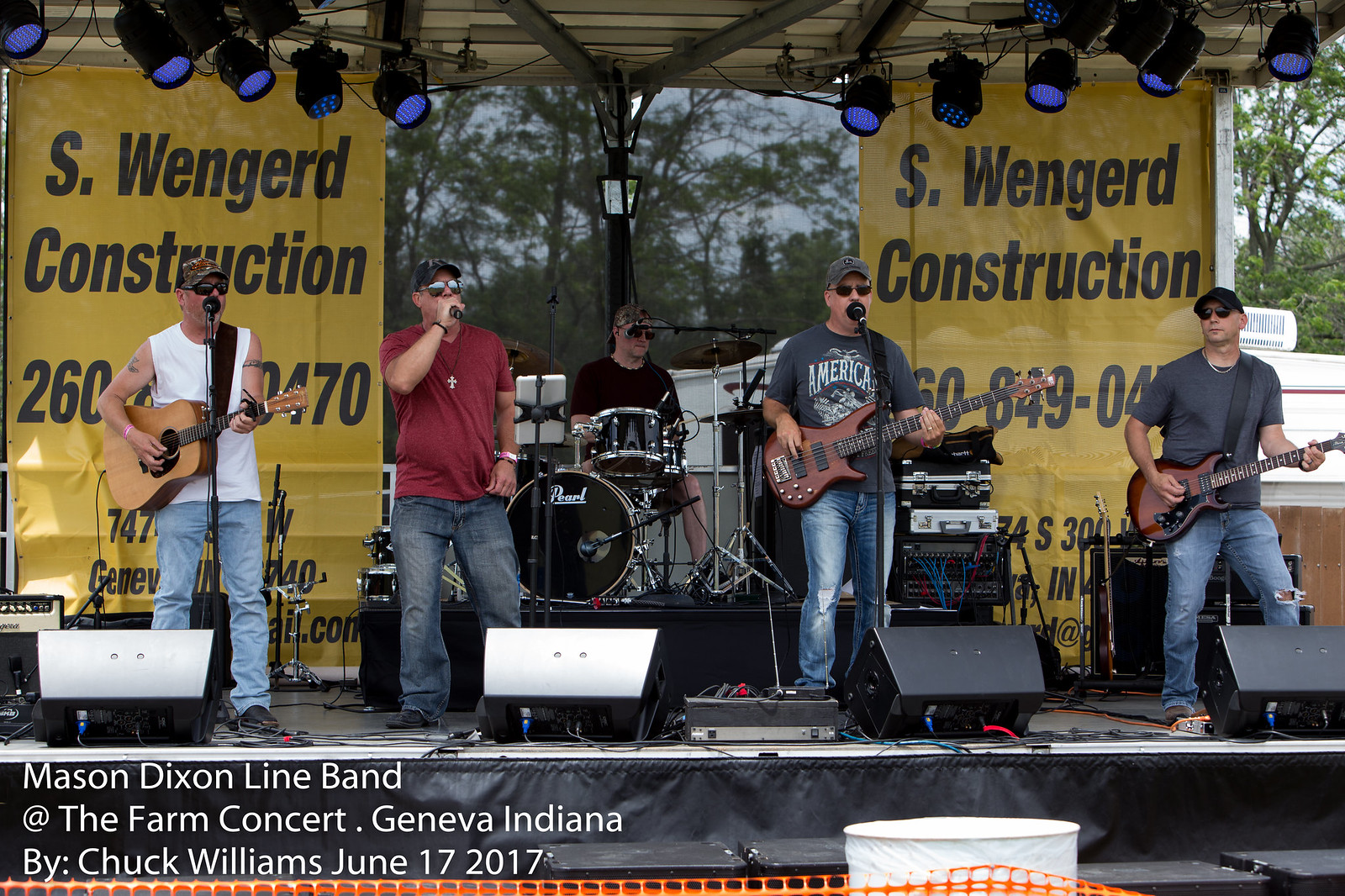The rectangular photograph captures the Mason-Dixon Line Band performing at the Farm Concert in Geneva, Indiana, by Chuck Williams on June 17th, 2017. The backdrop consists of yellow banners with black print reading "S. Wengerd Construction" along with a partially obscured phone number, nestled against a grayish blue sky and a veil of trees. The band, bathed in the glow of blue stage lights, consists of five members all adorned in sunglasses and hats.

From the left, the first musician sports a white sleeveless t-shirt, blue jeans, and camel hat, strumming an acoustic guitar while singing into a microphone. Next to him, the presumed lead singer, clad in a red t-shirt, blue jeans, and another camel hat, passionately engages the audience with his vocals. At the center, the drummer, in a black t-shirt and camel hat, commands a black and chrome drum set. To his right, the bassist wears a grayish baseball cap, a grayish black t-shirt emblazoned with "America," and blue jeans, contributing both instrumental and vocal elements. The final band member on the far right, dressed in a dark baseball cap, gray t-shirt, and blue jeans, plays the electric guitar.

A faint orange snow fence marks the boundary between the band and the unseen audience, capturing the essence of this lively outdoor performance. The detailed identifiers and cohesive stage setup highlight the event's vibrant atmosphere and the band's dynamic presence.